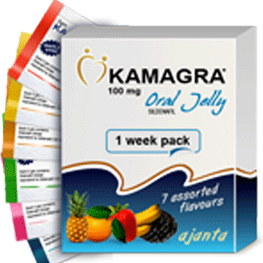This color photograph depicts a product called Kamagra 100mg Oral Jelly. The packaging, which is a white box with a blue wave-like design at the bottom, prominently displays the text "Kamagra, 100 milligram, oral jelly, one week pack, seven assorted flavors." The lower section of the box features images of various fruits, including a pineapple, an orange, an apple, some bananas, and a blackberry, representing the different flavors available. To the left of the box, there are six visible packets, each with a distinct color stripe—red, orange, yellow, green, pink, and blue—indicating the assorted flavors contained within the box. The professional layout and detailed design of the packaging emphasize its purpose as an oral jelly product, aimed at alleviating erectile dysfunction symptoms in men.